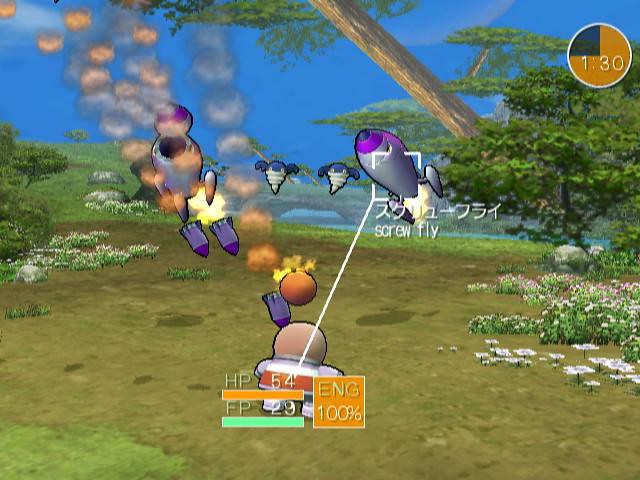In this detailed screenshot from a video game, the scene is set in an open field with a mix of brown and light brown ground, accented by patches of green grass and various flowers. Notably, the bottom left corner has a green patch, while the right side of the field blooms with white and purple flowers interspersed with green bushes. To the left, additional flowers, grassy patches, and bushes are visible. The central character is a short, animated figure with a circular head, dressed in a white and orange suit. Onscreen statistics for this character display HP at 54, FP at 29, and ENG at 100%, with corresponding orange and green bars for HP and FP, and an orange square indicating full energy. The character appears to be under attack, with blue rockets and an orange circular bomb directed at them. In the backdrop, trees line the right-hand side, a hill rises on the left, and a blue sky frames a circular clock marked as 1:30, predominantly shaded orange with a dark blue quarter and a white outer ring. Smoke and fire trail some of the descending bombs, adding to the chaotic atmosphere.